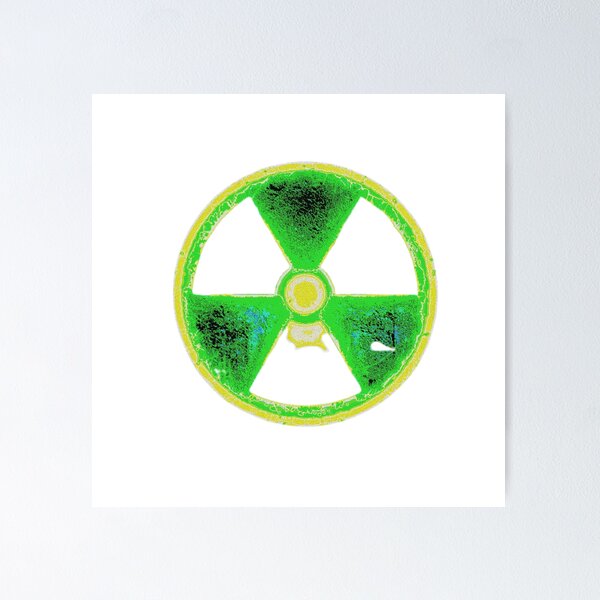The image depicts a graphical illustration situated on a square piece of white watercolor paper, framed by a wide, light gray matte. Centrally featured is a series of concentric circles: the outer circle is a goldish yellow, while the inner circle is green. At the 12, 5, and 9 o'clock positions, the green circle includes fan-like white triangles. There are six alternating triangular shapes radiating from the center, with green triangles showing dark and black spots, and white triangles. The design, reminiscent of a modified radioactive symbol, has a faded, aged appearance, suggesting the colors have rubbed off in places. The inner circle's center is a darker yellowish gold, with the top of the 6 o'clock white triangle touched by this color.